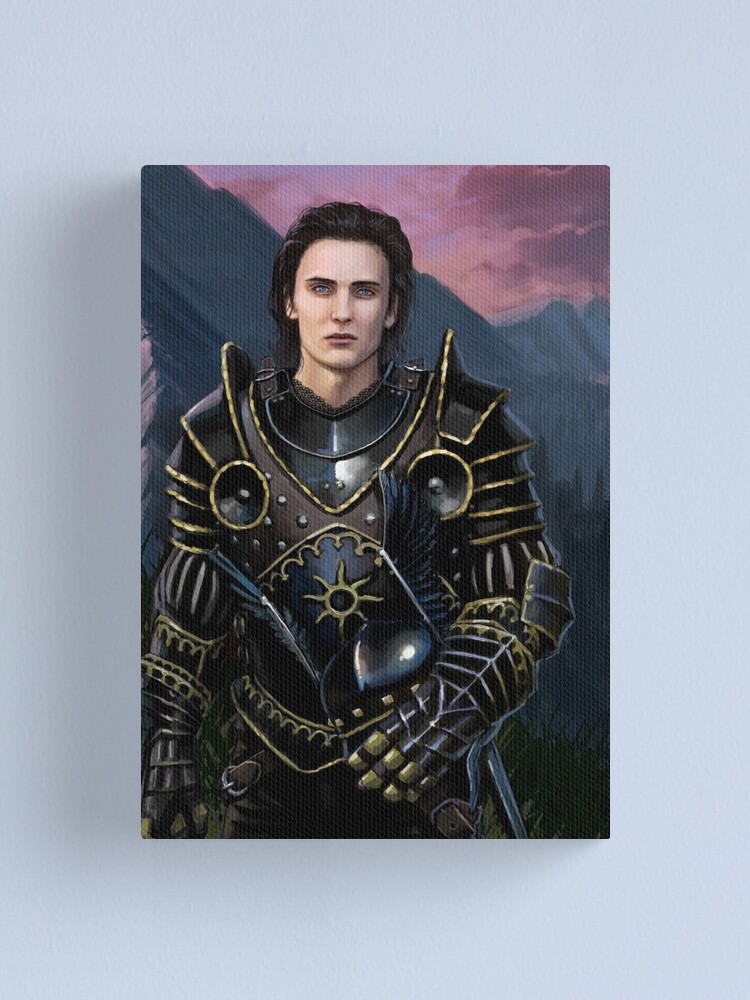This image depicts a young knight in elaborate black armor with gilded gold edges and intricate details on the shoulder plates and gloves. His pale skin contrasts sharply with his long, dark hair, which is slicked back to reveal his symmetrical face, piercing blue eyes, and strong jawline. Holding his ornately designed helm in his gauntleted left hand, the helm features feathers, two eagle wings, and horns. The centerpiece of his breastplate is a sun emblem intricately lined in gold. A sheathed sword hangs by his left hip. He stands against a dramatic backdrop of gray and black mountains, under a purple-pink sky with ominous red clouds above, with hints of a forest and grass below his feet. The artwork, although slightly out of focus, captures the essence of a serious and formidable fantasy warrior.